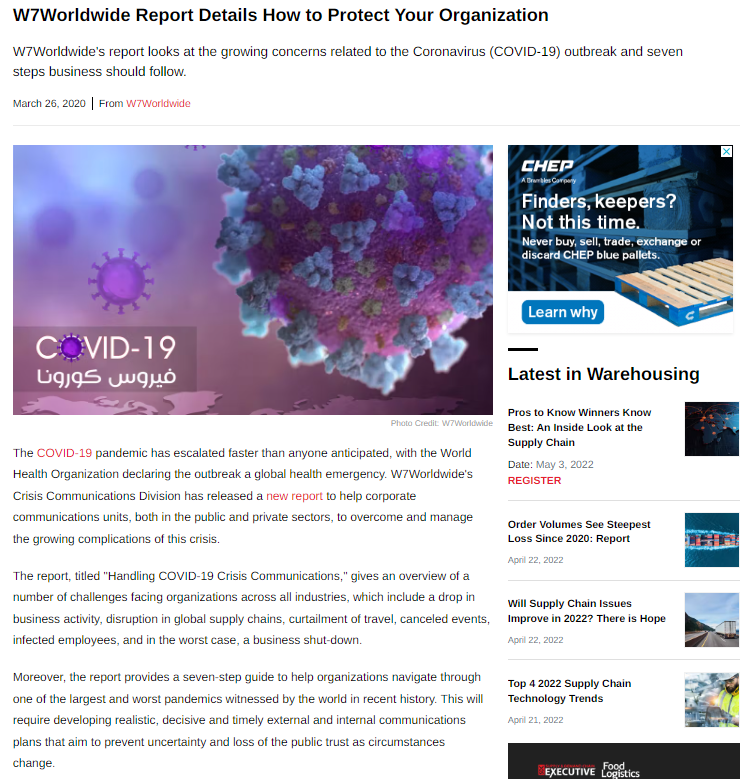Screenshot on a white background featuring details from W7 Worldwide's report titled "Protecting Your Organization". The report, highlighted in red, addresses the mounting concerns related to the coronavirus (COVID-19) outbreak, focusing on seven integral steps businesses should follow. Dated March 26, 2020, from W7 Worldwide, the image includes a visual representation of the COVID-19 virus with the text "COVID-19" prominently displayed in red. Beneath the image, additional text appears in a different language. The report underscores how the COVID-19 pandemic has escalated rapidly, prompting the World Health Organization to declare it a global health emergency. W7 Worldwide's crisis communications division has issued this new report, marked in red, aimed at assisting corporate communications teams in both the public and private sectors to navigate and manage the complexities of the crisis. On the left side of the screenshot, there is a section titled "Latest in Warehousing," featuring four articles.